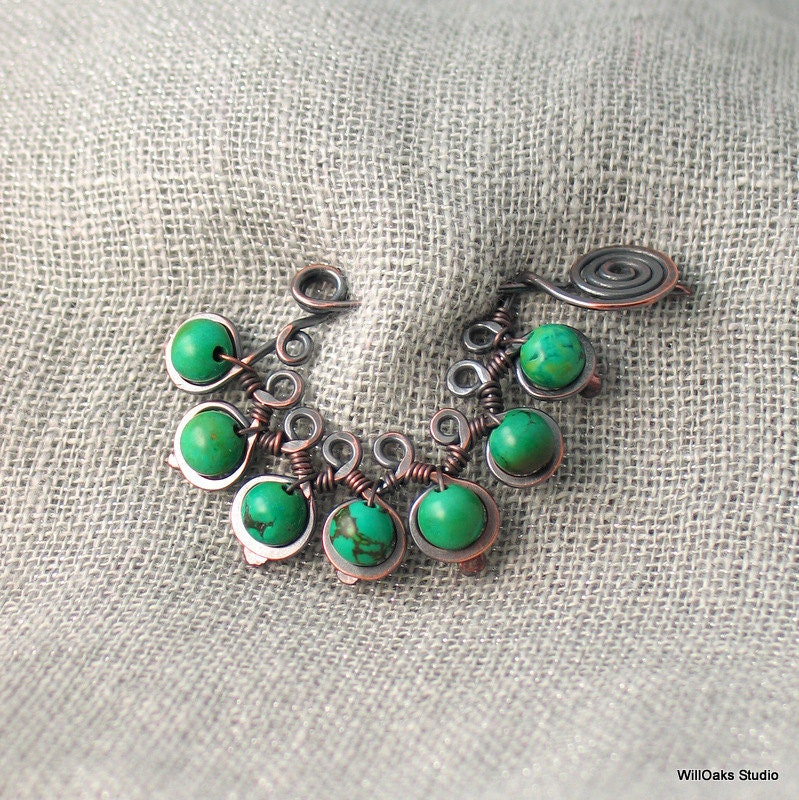This color photograph showcases a beautifully crafted piece of copper jewelry, intricately displayed on a beige burlap backdrop. The jewelry, likely a brooch or pin, features a twisting and spiral pattern that binds seven small, pea-sized green stones, some with black veining. Each green stone is encased in a loop of metal, creating a harmonious and aesthetic design. The right side of the piece culminates in an elegant spiral, while the left side is affixed through the burlap with a pin, typical of lapel pins. The artistry is further emphasized by wrapped wire throughout the design, adding ornate decoration. The craftsmanship is credited to WillOaks Studio, as indicated by the writing in the bottom right corner of the photograph.